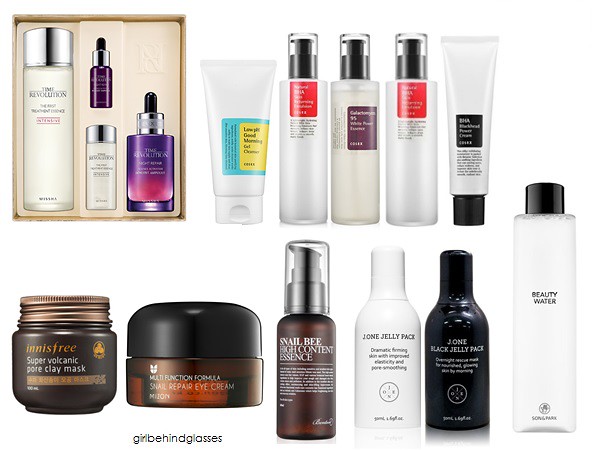This stock photo showcases an array of beauty products, meticulously arranged, possibly for promotional purposes on a retail website. Dominating the upper left corner is an elegant gift box containing four distinct bottles. Among them, the most prominent bottle, positioned far left, is labeled "Time Revolution." This bottle is pure white with a sleek silver cap, exuding a minimalist elegance. Adjacent to it, a smaller bottle captures attention with its striking purplish-red hue topped by a stainless steel cap and black dropper. A larger counterpart of this bottle is located to the bottom right of the gift box, maintaining the same luxurious design.

Beneath, at the bottom center of the image, sits a product called "Super Volcanic Pore Clay Mask" from the brand Innisfree, denoted by its earthy tones and sturdy appearance. To its immediate right is another intriguing item – a multifunctional "Snail Repair Eye Cream," although slightly obscured by reflection, hinting at its potential to rejuvenate delicate skin.

Continuing rightward, a bottle marked "Snail Bee High Content Essence" stands tall, promising intensive nourishment. The sequence proceeds with the "J1 Jelly Pack," followed by a similar black bottle labeled "J1 Black Jelly Pack," each emphasizing unique skincare benefits. Concluding the impressive lineup, on the far right, is a pristine white bottle titled "Beauty Water," capped with a stark black lid, offering a final touch of refinement to the diverse collection.